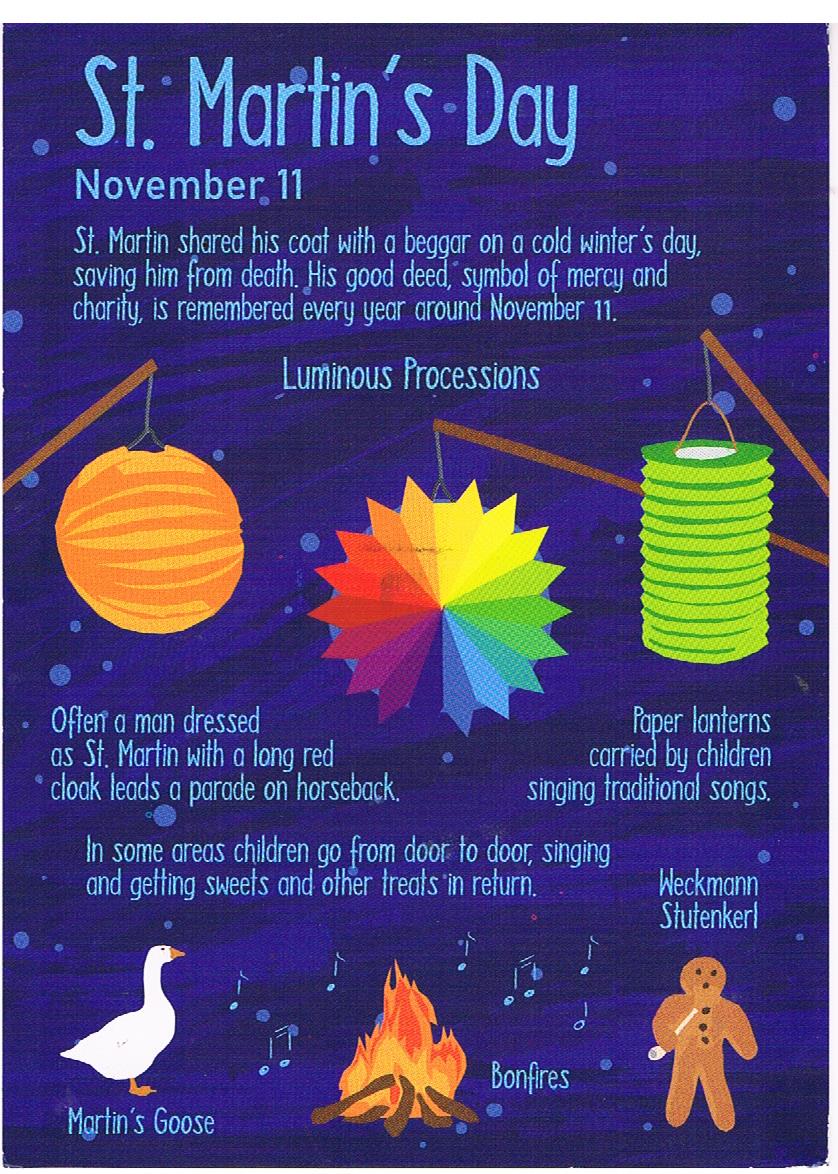The vertically aligned rectangular image features a predominantly blue background, with varying shades of medium and dark blue interspersed with light blue dots resembling bubbles. At the top of the image, "St. Martin's Day" is written in light blue text, left-aligned, followed by the date "November 11th." Below this, in smaller blue text, is the following description: "St. Martin shared his coat with a beggar on a cold winter's day, saving him from death. His good deeds, a symbol of mercy and charity, are remembered every year around November 11th."

Centered beneath this text, the words "Luminous Processions" are displayed. Below this are illustrations of paper lanterns: on the left, a brown pole is holding a round orange lantern; in the center, a brown pole is holding a multicolored star-shaped lantern; and on the right, another brown pole is holding a green cylindrical lantern. The text underneath the orange lantern reads: "Often a man dressed as St. Martin, with a long red cloak, leads a parade on horseback." Below the green cylindrical lantern, it states: "Paper lanterns carried by children singing traditional songs." The next line notes: "In some areas, children go from door to door singing and receiving sweets and other treats in return."

Along the bottom of the image are three smaller pictures: on the left, an illustration of a white goose labeled "Martin's Goose," in the center, an image of a bonfire labeled "Bonfires," and on the right, a brown gingerbread man labeled "Weckman Student Curve."